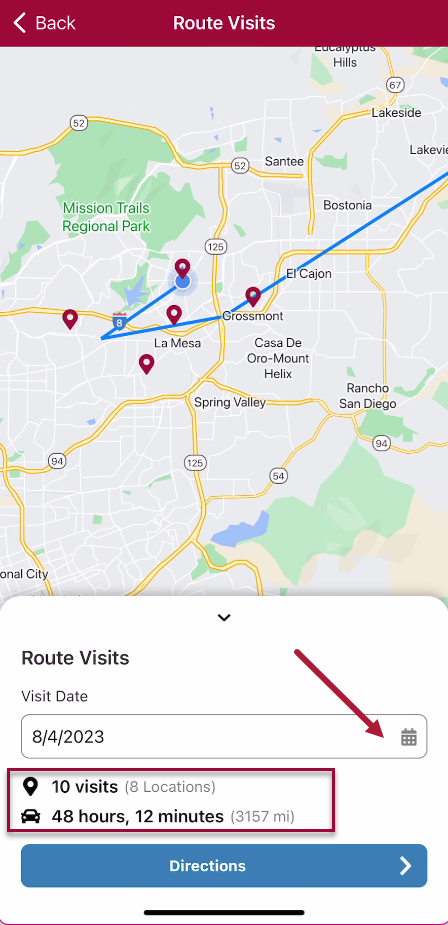This is a detailed screenshot of a GPS navigation system, providing an overview of a recent journey. In the upper left-hand corner, there is a "< Back" button displayed in white. The central portion of the screen prominently features the label "Route Visits."

A red bar spans the top of the image, beneath which a map is shown, detailing several key landmarks and cities. Located in the upper left-hand corner of the map is Mission Trails Regional Park. To the upper right, Lakeside can be seen. The bottom right of the map highlights Rancho San Diego, while Spring Valley is situated to the left of it. Grossmont is marked at the very center of the map.

The map also includes other areas centrally positioned such as El Cajon, Bostonia, and Santee. Major highways labeled on the map are 94, 125, 54, 52, and 67. There are several pins marking various points along the route, indicating significant stops or destinations.

The journey appears to follow Highway 8, passing notable areas like La Mesa, Grossmont, and El Cajon, and proceeds in a northeast direction. At the bottom of the app, detailed visit statistics are provided. The “Visit Date” is listed as 8/4/2023. Additional metrics include "10 visits," "8 locations," "48 hours and 12 minutes," and a total distance of "3,157 miles." A right-pointing arrow is also located at the lower right corner of the screen.